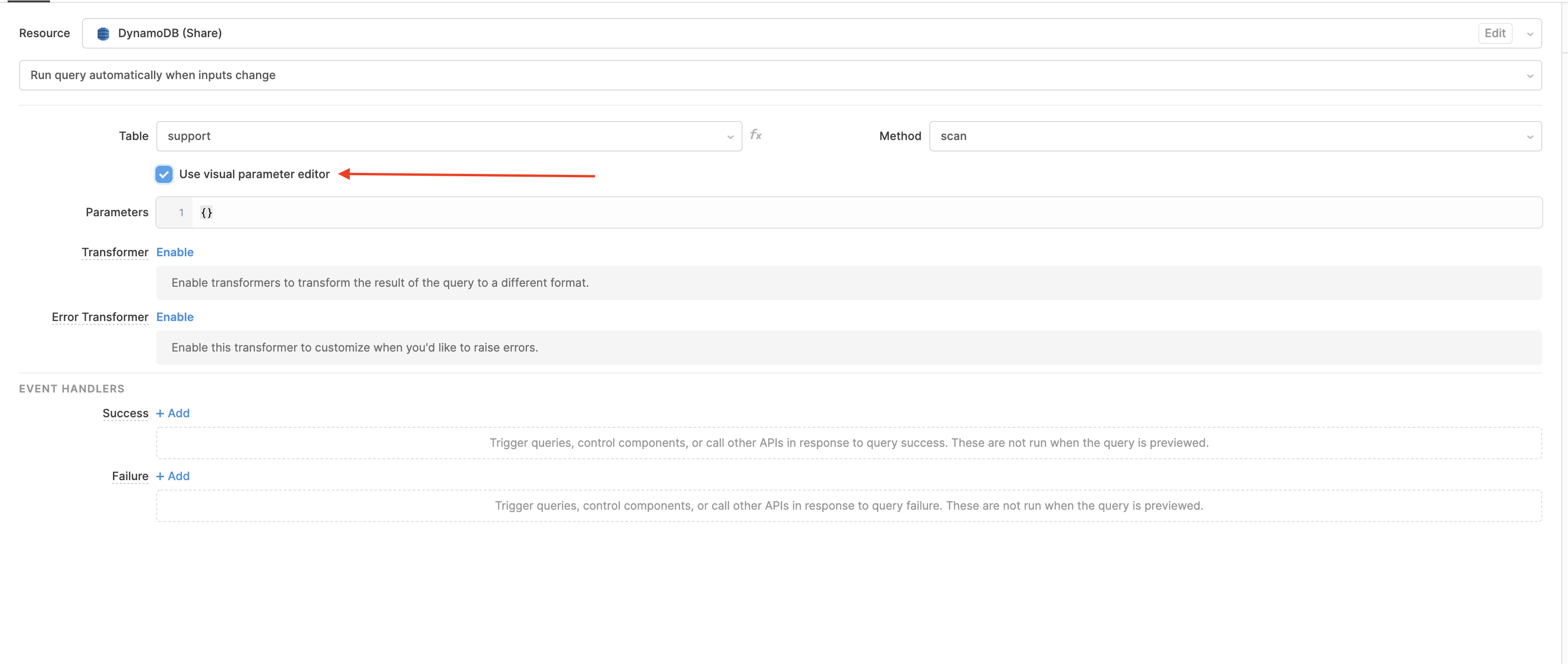Screenshot Description:

The image appears to be a partial screenshot of a software interface, primarily set against a white background. At the top, there is a main menu heading that includes the words "Resource" followed by a vertical line and something resembling "Dynamic OS" or "Dynamo OS Share". Below this heading, there is a phrase that appears to say "Scan query automatically when inputs change." 

Inset within the main interface, there is a table featuring dropdown options labeled "Support" and "Method Scan." 

Further down, another inset section contains a blue rectangle with a prominent white check mark inside it. This rectangle bears the text "Use Visual Parameter Editor," with a long red arrow pointing to it from left to right, clearly drawing attention to this feature. 

Below this highlighted feature, there is a section labeled "Parameters," which lists "Transformer Enable" followed by some other unreadable text. Additionally, the section includes "Error Transformer Enable" followed by more unreadable text. 

At the bottom of the visible interface, there are options for "Event Handlers," which include buttons labeled "Success + Add" and "Failure + Add." On the far right side of the image, there is more text that is too small and faint to read clearly. 

In summary, the screenshot captures a complex software interface, but its small size and fine print make it challenging to discern all details clearly. [Note: The difficulty in reading and describing the image emphasizes the need for larger and clearer visuals for effective description.]